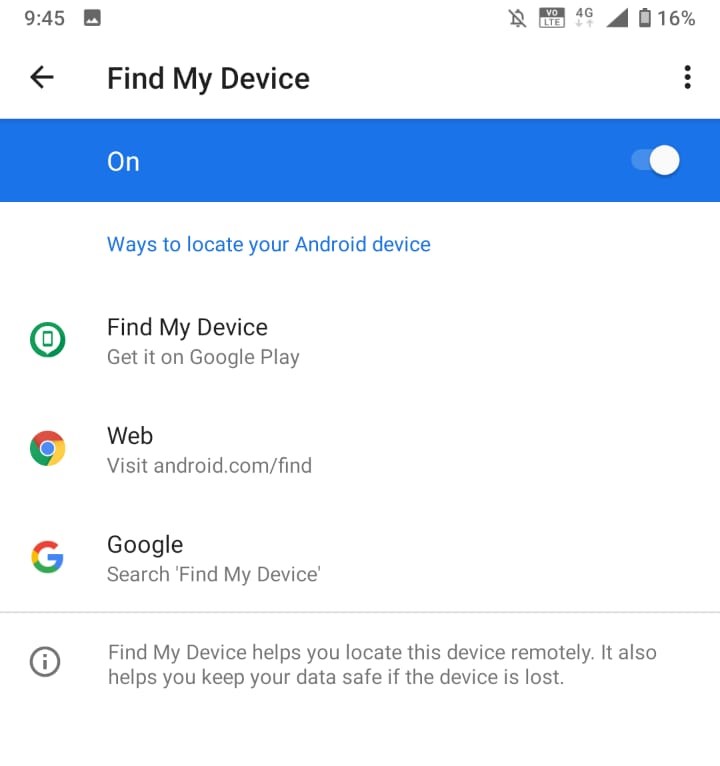The screenshot depicts a smartphone screen with key details about the phone’s status and a specific application setting. In the upper left corner, the time is displayed as 9:45. To the right, the battery icon indicates it is at 16% and the phone is connected to a 4G network. Below this, there is an icon resembling a calendar, followed by a left-pointing arrow.

On the main part of the screen, the text reads “Find My Device” next to a blue rectangular area containing the word "ON." To the right of this area, a toggle switch is enabled, indicated by its white color. 

Underneath this, a section titled “Ways to locate your Android device” is present, listing three options:

1. A circular icon with a rectangle inside it, indicating the “Find My Device” app available on Google Play.
2. Another circular icon featuring bands of red, yellow, green, and blue, guiding the user to visit android.com/find via the web.
3. The multicolored "G" of Google, suggesting using Google Search to find the device.

At the bottom left of the screen, a small circular icon with a lowercase "i" draws attention. Accompanying text explains that the "Find My Device" feature assists in locating the device remotely and securing data if the device is lost.